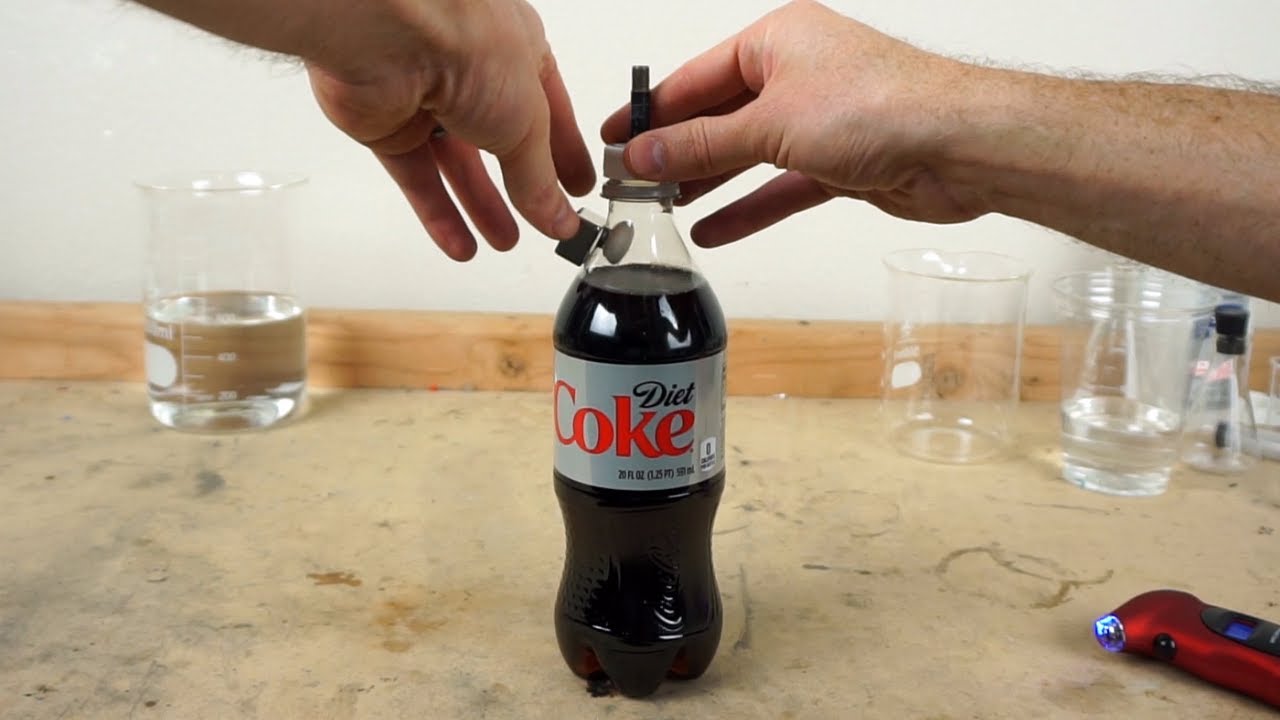The image features a 20 fl oz bottle of Diet Coke positioned on a beige surface with a tan wooden border, set against a white wall. The bottle, which is full of dark liquid, has a gray label with "Diet" written in black and "Coke" in red. The words "20 fl oz" and "zero calories" are also visible on the right side of the label. A black tube sticks out of the white cap of the bottle. Two human hands are interacting with the setup: the right hand is gripping the white cap, while the left hand is holding a square silver metal cube, possibly a magnet, close to the top of the bottle. Additionally, clear glass beakers containing a clear liquid are situated in the background. This setup suggests a Mentos and Diet Coke experiment.